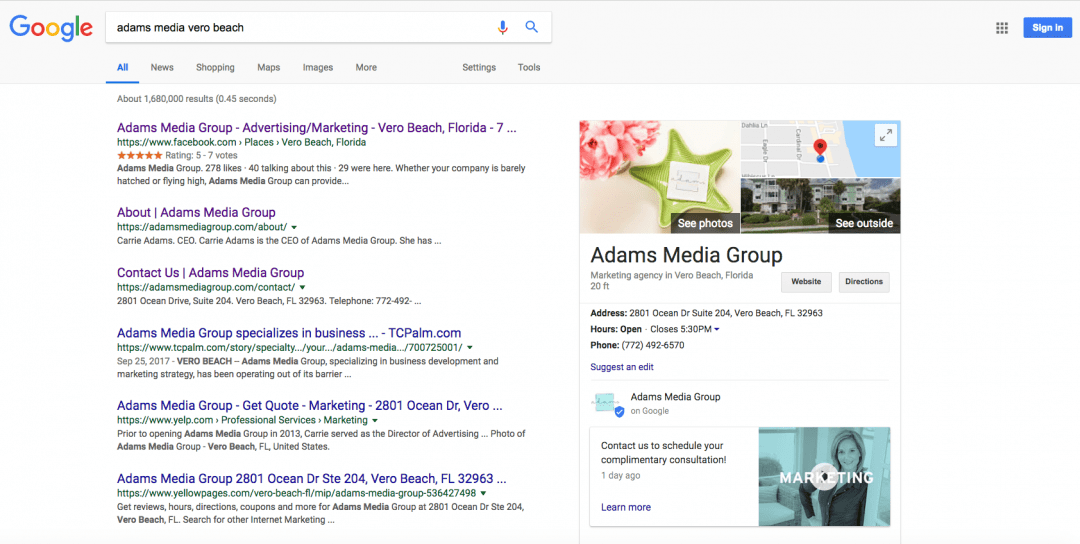Here is a detailed, cleaned-up description of the image:

---

The image displays a Google search results page. The interface is in standard mode with a white background and a light gray top bar. In the upper left corner, the multicolored Google logo is prominently visible. To the right of the logo is the white search bar containing the search query "adams media vero beach" typed in lowercase black text. Adjacent to the search bar, there is a microphone icon followed by the magnifying glass search icon. On the far right, the top bar features a grid icon with three rows of three boxes each and a blue "Sign in" button with white text.

Below the search bar, there are various search filter options: All, News, Shopping, Maps, Images, More, Settings, and Tools. The "All" option is selected, highlighted in blue, and underlined. Directly beneath these options, the page indicates that there are about 1,608,000 results, which were fetched in 0.45 seconds.

The main section of the page displays six website listings related to "Adams Media Vero Beach." The first three listings have purple titles, implying that they have been previously clicked, whereas the last three are blue.

1. **First Listing:**
   - **Title:** Adams Media Group Advertising-Marketing Vero Beach, Florida
   - **URL:** Facebook.com page specific to Vero Beach, Florida
   - **Ratings:** 5 orange stars from 5 to 7 votes
   - **Description:** Adams Media Group has 278 likes, with 29 people having checked in. The statement provided is incomplete: "Whether your company is barely hatched or flying high, Adams Media Group can provide..."
   - **Visuals:** To the right of this listing, there are three images:
     - A white table with a bouquet of pink flowers and a green star, along with the text "See photos."
     - A map featuring gray land, a red pinpoint, and a blue ocean.
     - An exterior shot of buildings with the label "See outside."
   - **Additional Information:**
     - **Website Button:** Gray button with black text "Website"
     - **Directions Button:** Gray button with black text "Directions"
     - **Address:** 2801 Ocean Drive, Suite 204, Vero Beach, Florida 32963
     - **Hours:** Open until 5:30 PM, with an arrow indicating more hours are available.
     - **Phone:** 772-492-6570
     - **Note:** There is an option to suggest an edit, as well as details about the firm's Google validation with a blue shield and white checkmark.
     - **Video Thumbnail:** A promotional video with a blue filter featuring a smiling woman and the text "MARKETING" with a play button.

2. **Remaining Listings:**
   - **Second Listing:** "Carrie Adams, CEO of Adams Media Group" with a specific URL for contact at adamsmediagroup.com.
   - **Third Listing:** "Contact us, Adams Media Group," leading to a contact page on their official website.
   - **Fourth Listing:** An article titled "Adams Media Group specializes in business development and marketing strategy" from tcpalm.com, dated September 25, 2017.
   - **Fifth Listing:** "Get Quote Marketing" related to Adams Media Group with an address mention.
   - **Sixth Listing:** From Yellow Pages, providing information about Adams Media Group, including their address, review hours, directions, and coupons.

The search results provide comprehensive details about Adams Media Group's presence, from social media and official website listings to external articles and business directory entries.

---